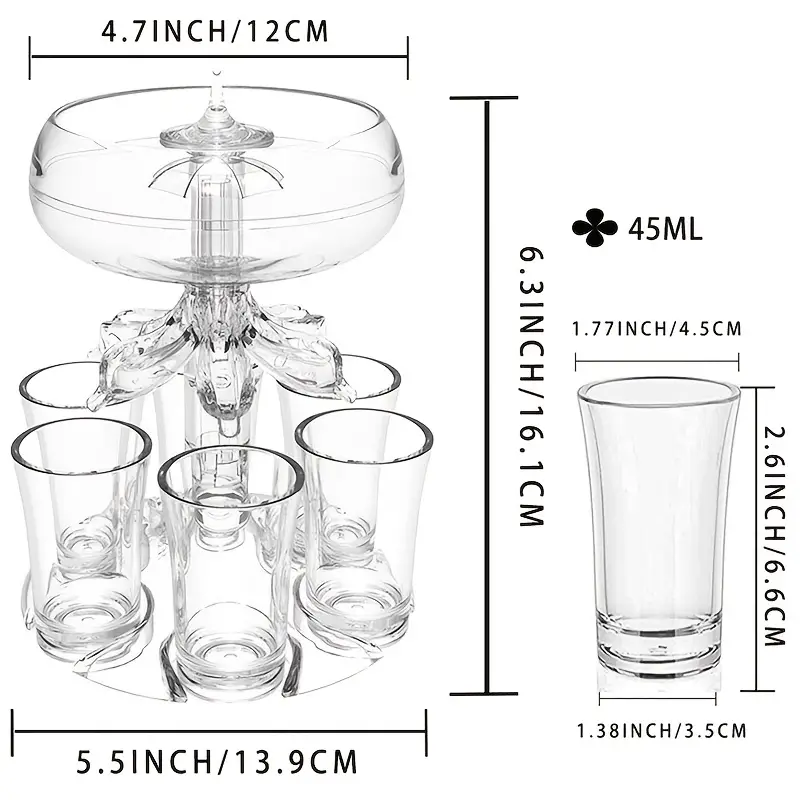This image displays a detailed diagram of a drink serving set, which resembles a product for sale on Amazon. The centerpiece is a clear bowl, measuring 4.7 inches (12 centimeters) in diameter across the top, mounted above six evenly spaced spouts. These spouts are designed to dispense liquid simultaneously into six glasses positioned beneath them. The ensemble stands 6.3 inches (16.1 centimeters) tall. The width across the base, where the glasses are arranged, is 5.5 inches (13.9 centimeters). Each shot glass in the set has a top diameter of 1.77 inches (4.5 centimeters), a height of 2.6 inches (6.6 centimeters), and a base diameter of 1.38 inches (3.5 centimeters). The glasses can hold up to 45 milliliters of liquid. The measurements are prominently displayed in black text on a clean, monochromatic background, ensuring clarity.